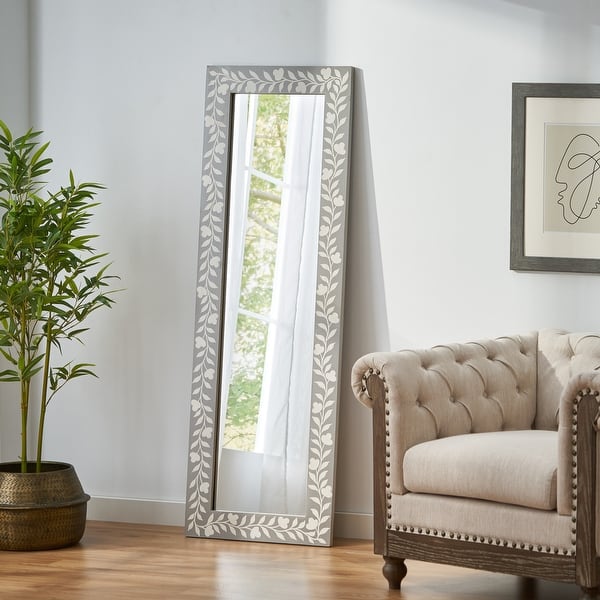This color photograph captures a bright and airy room with clean white walls and a polished light brown hardwood floor. On the left side of the image, there's a copper or bronze planter housing a palm-style tree with thin stalks and medium green leaves. Centered in the room, leaning against the wall, is a tall, rectangular mirror with a silver frame adorned with a floral and leaf pattern. The mirror reflects a window with billowy white curtains, adding to the room's open feel. To the right, a plush, tufted armchair with high arms and a nailhead trim stands, featuring a light gray or beige fabric and a wooden frame and legs. Above the chair, a framed abstract line drawing in a dark gray or brown frame adds an artistic touch. The overall scene combines elements of warmth and elegance, creating a comfortable, stylish interior.